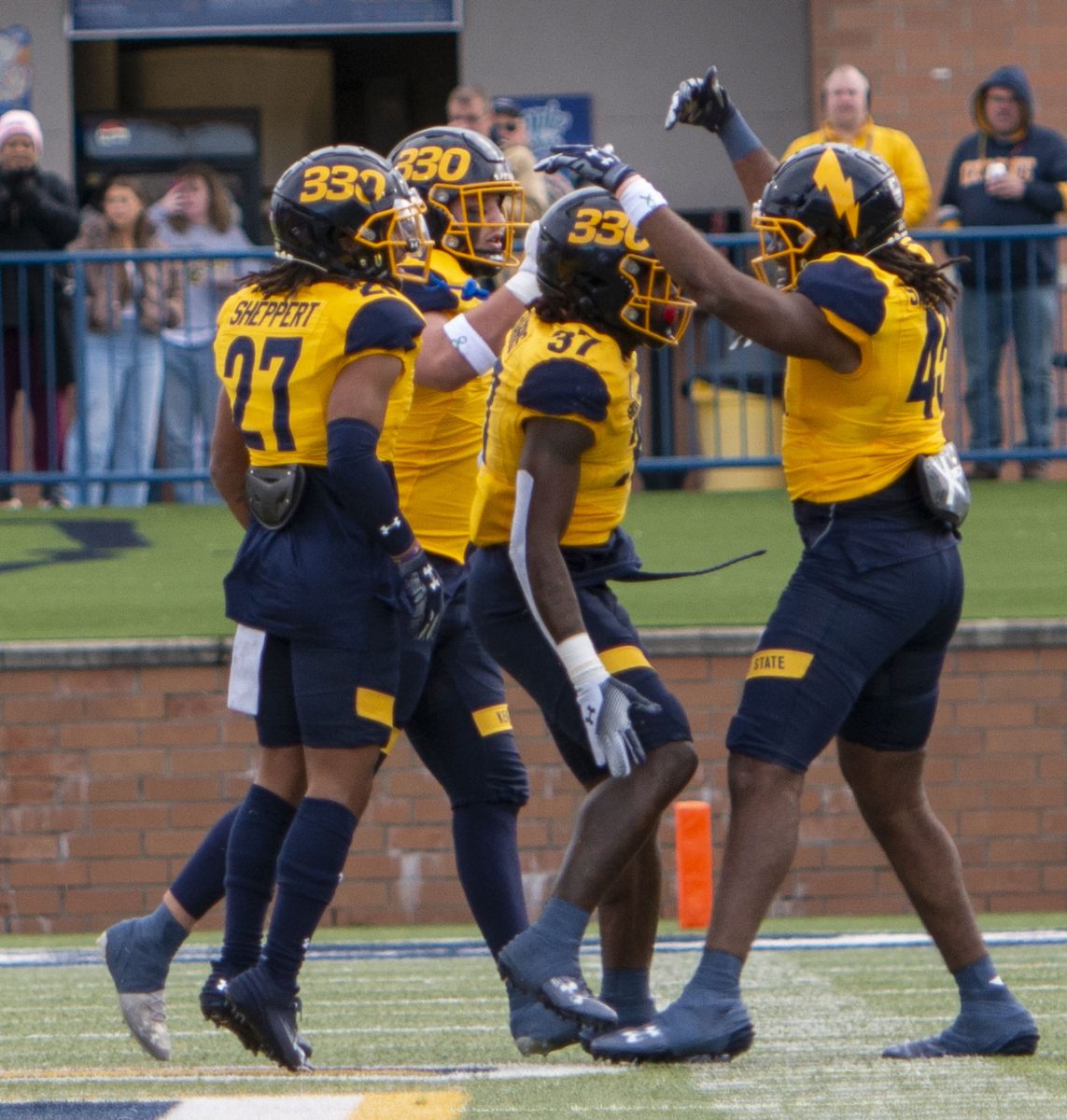In the image, set on a partly cloudy day, four football players are captured mid-celebration on a field adorned with visible yard lines. These athletes, attired in vibrant yellow jerseys, black helmets marked with the number 330, and black cropped pants, embody a diverse group with African-American and white teammates. The central focus is on one player with outstretched arms, seemingly ready to embrace another, who has his arms lifted as if prepared for a hug. One of the athletes, notable for his hair peeking out from under his helmet, adds dynamic energy by leaping into the air. In the background, a short red brick wall with a grassy verge forms a boundary, beyond which spectators can be seen enjoying the game. This snapshot vividly captures the exuberant moment of triumph and camaraderie on the football field.